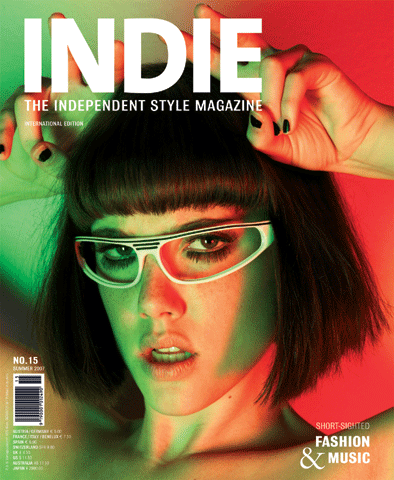The cover of the 15th edition of Indie, the Independent Style Magazine, released in November 2017, features a close-up portrait of a white woman sporting a short bob haircut and fringe bangs that rest just above her eyebrows. Her eyes are accentuated with heavy eye makeup, including eyeshadow and mascara, and she wears large, retro-style eyeglasses with wide eyepieces that have two lines in the centerpiece. Her expression appears somewhat unimpressed, with her lips slightly parted as she gazes directly at the camera. She raises her hands above her head, forming a gesture that resembles either peace signs or bunny ears with her first two fingers. Her black-painted nails add to her striking look. The backdrop transitions from green on the left to red on the right, casting warm, vibrant hues over her face. At the top, "Indie, the Independent Style Magazine" is written in white font, and at the bottom right, the phrase "Short Sighted Fashion in Music" is also displayed in white font. The bottom left corner includes additional information about the contents of the magazine and barcodes.